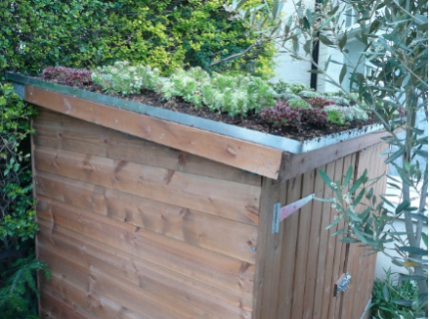The image captures a serene outdoor scene centered around a substantial wooden planter, likely a DIY project, crafted from blonde-colored wood. The planter notably features horizontal wood paneling with a small hinged access door on its front side, designed to easily manage the interior. A metal trim adorns the top of the planter, containing a variety of thriving plants, which appear to be vegetables rather than flowers. Among the predominately light green foliage are a few deep burgundy shrubs. In the backdrop, there is a lush, bushy green bush to one side and a unique bluish-green tree on the other, providing a natural, tranquil setting for this impressive, yet functional, planter display.